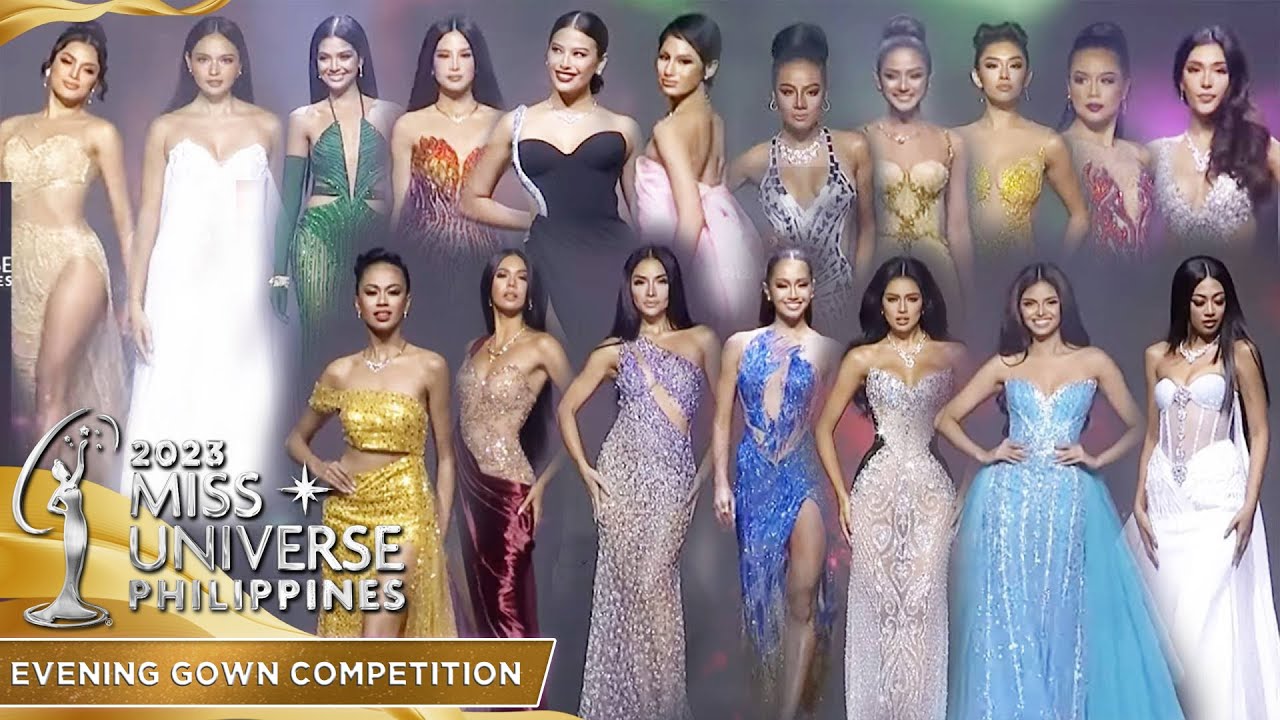This is an image of the 2023 Miss Universe Philippines Evening Gown Competition contestants. The text "2023 Miss Universe Philippines" appears in a shiny silver font at the lower left-hand corner, accompanied by a silver statuette icon, with "Evening Gown Competition" written beneath it. The contestants are arranged in two rows, with 11 women in the back row and 7 in the front row. They are all dressed in a variety of elegant evening gowns that span a wide spectrum of colors including cream, white, gold, green, yellow, black, pink, red, purple, and blue. The gowns are adorned with sequins and beading, showcasing different styles such as strapless, one-shoulder, and long-sleeved, and include intricate designs from flowy ball gowns to more form-fitting cuts. Each contestant wears her hair in elaborate styles, either slicked back, straight, or styled down, and accessorizes with necklaces, earrings, and the occasional bracelet. They smile or make sultry expressions against a gray background highlighted with purple and green light splotches. The women's overall appearance exudes glamour and sophistication, capturing the essence of the competition.